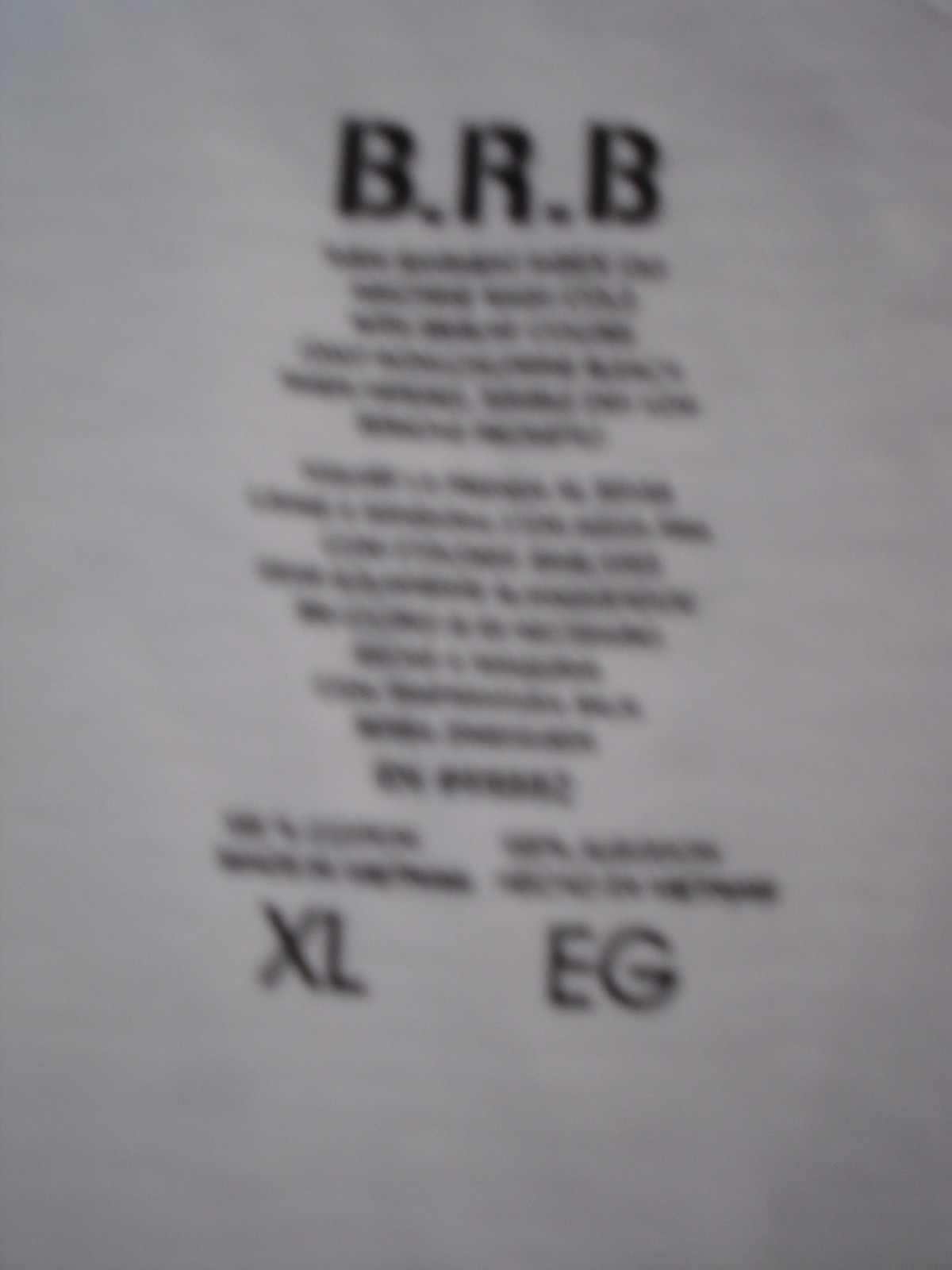The image is a blurry, dimly-lit photograph of the inside of a white t-shirt, showing a screen-printed tag in black text. The logo "B.R.B." is prominently displayed at the top in bold, uppercase letters. Below the logo, the sizing information "XL" and "EG" is shown in large text on the left and right sides, respectively. The rest of the text, likely containing washing instructions and fabric composition details in both English and Spanish, is small and completely blurred, making it illegible. The shirt is open in a way that casts a shadow over part of the tag, adding to the difficulty of reading the finer print.